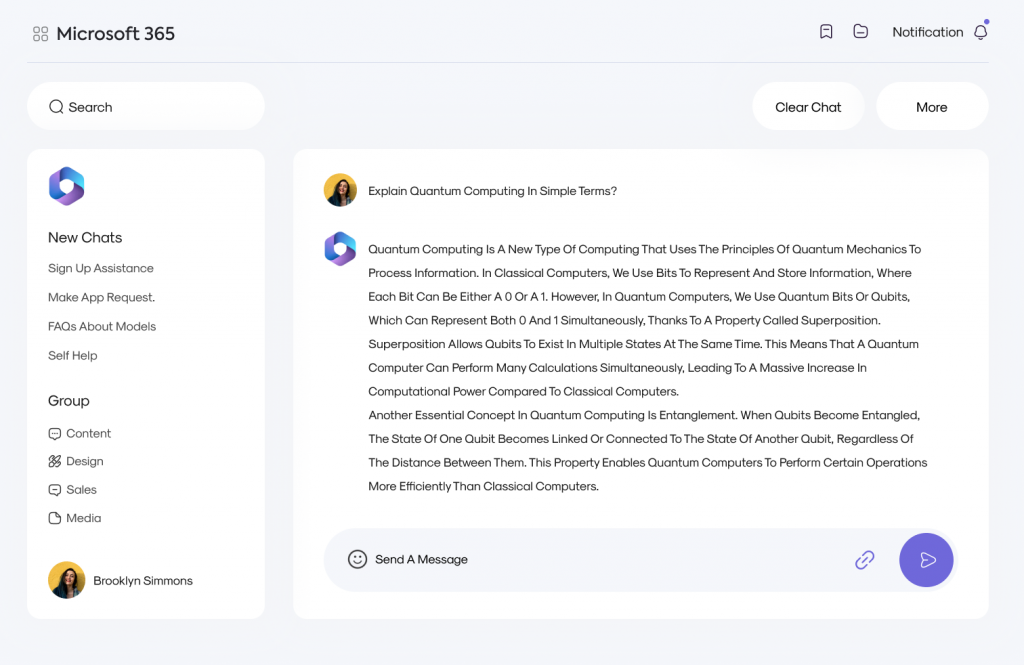The screenshot captures a webpage from Microsoft 365. The background is light gray. At the top left corner, inside a small square, there are four smaller squares forming the Microsoft logo next to the text "Microsoft 365" in large, black, capitalized font.

To the top right, there are some icons, including a notification bell with a blue dot indicating new notifications. Below this, a white search bar features a gray magnifying glass icon and the word "Search" in gray text. Further to the right are options labeled "Clear chat" and "More."

On the left side of the screenshot, a sidebar with a blue and purple design includes various menu items: "New chats," "Sign up assistant," "Make app request," "FAQs about models," "Self-help," "Group," "Content design," "Sales," and "Media." Below these options, the name "Brooklyn Simmons" is displayed next to a profile image set against a gold circular background.

In the center of the image, a white background showcases a repeated display of Brooklyn Simmons' profile image. Below it, a text prompt asks to "Explain quantum computing in simple terms." The response, originating from an icon within the blue and purple design, begins to elaborate: "Quantum computing is a new type of computing that uses principles of quantum mechanics to process information," and further details are provided in the response.